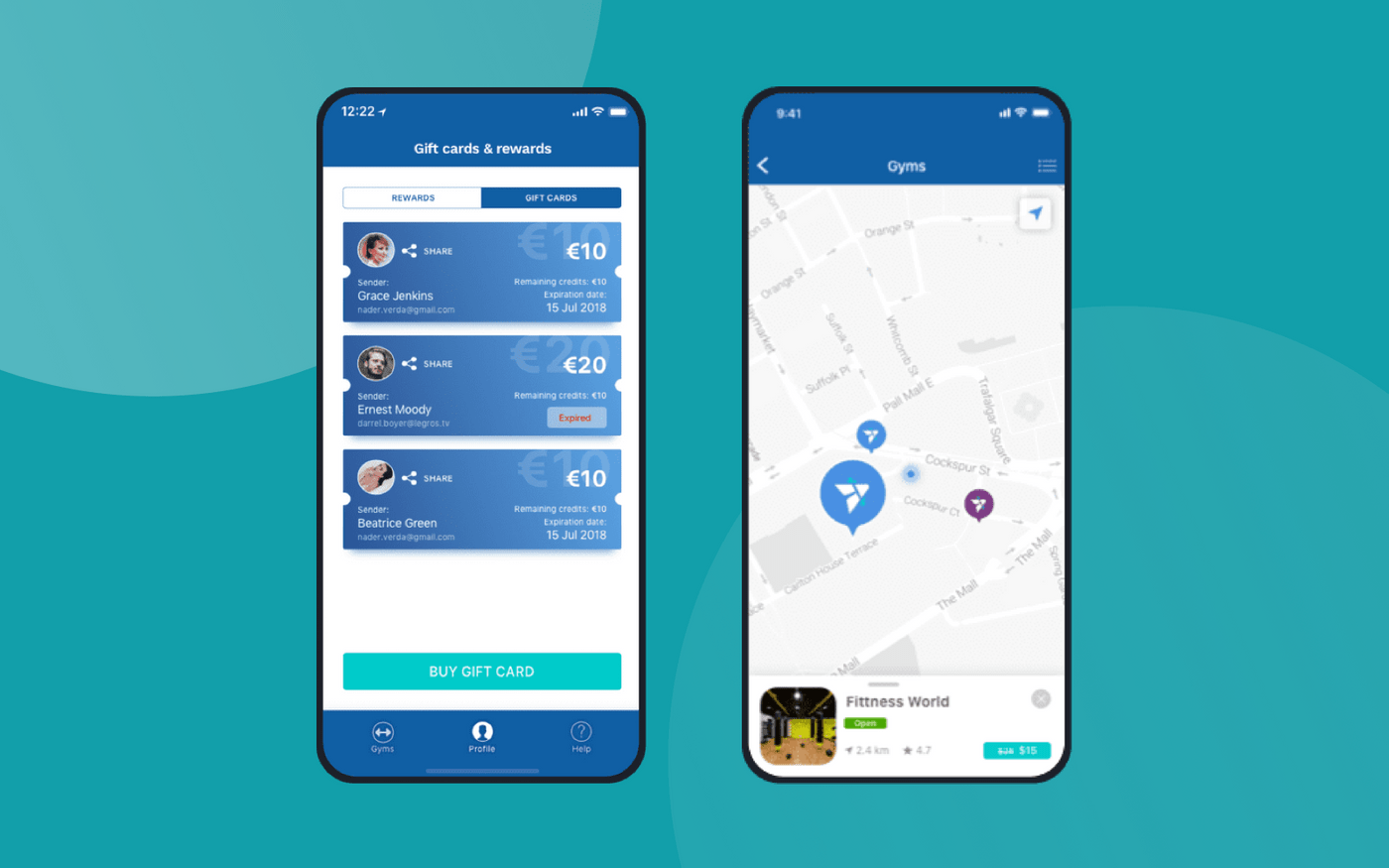The image features a screenshot of a gift and rewards program displayed on two different phones, set against a blue background.

**Left Phone Display:**
The screen presents two sections of the rewards program: "Rewards" and "Gift Cards", with the "Gift Cards" option currently highlighted in blue. The display lists three gift cards:
1. **Gift Card 1**:
   - **Sender**: Grace Jenkins
   - **Value**: £10
   - **Remaining Credits**: £10
   - **Expiration Date**: July 15th, 2018
2. **Gift Card 2**:
   - **Sender**: Ernest Moody
   - **Value**: £20
   - **Remaining Credits**: £10
   - **Expiration Status**: Expired
3. **Gift Card 3**:
   - **Sender**: Beatrice Green
   - **Value**: £10
   - **Remaining Credits**: £10
   - **Expiration Date**: July 15th, 2018

At the bottom of the screen is a green button labeled "Buy Gift Card." Below this button are three additional buttons with blue backgrounds and white emblems:
- **Gyms** (left-hand side)
- **Profile** (middle)
- **Help** (right-hand side)

**Right Phone Display:**
The screen shows a map with various locations marked by symbols resembling flying notes, labeled "Gyms." A selected option on the map reveals "Fitness World" at the bottom of the screen, indicating the user’s interest in this particular location.

The dual phone display against the blue background provides a comprehensive overview of the gift and rewards program's interface and functionalities on both devices.